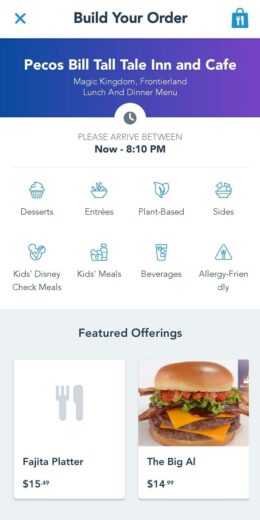A mobile screenshot of a delivery app, likely Uber Eats, displays a user interface for building a meal order. The screen is predominantly white with a vertical orientation, though the resolution is somewhat low. At the top of the screenshot, the header reads "Build Your Order," accompanied by a logo of a blue shopping bag adorned with a fork and knife, reinforcing the Uber Eats affiliation.

Below the header, a blue banner presents essential details: "Pecos Bill Tall Tale Inn and Café, Magic Kingdom, Frontierland, Lunch and Dinner Menu." It also specifies, "please arrive between now and 8:10 p.m."

Under the banner, there are several options and blue icons arranged in two rows of four each. From left to right, the categories are:

1. **Desserts** – represented by a cupcake icon.
2. **Entrees** – marked with a salad icon.
3. **Plant-Based** – illustrated with leaf icons.
4. **Sides** – possibly symbolized by a chicken icon.
5. **Kids Disney Check Meals** – showing an image of Mickey Mouse with a check mark.
6. **Kids Meals** – depicted with nuggets and a drink.
7. **Beverages** – shown as a glass icon.
8. **Allergy-Friendly** – featuring a triangle with a fork.

Beneath these categories is a section titled "Featured Offerings," highlighting items such as the "Fajita Platter" and "The Big Al." An image of a two-patty hamburger with cheese, bacon, tomato, and lettuce is visible, showcasing one of the featured items.